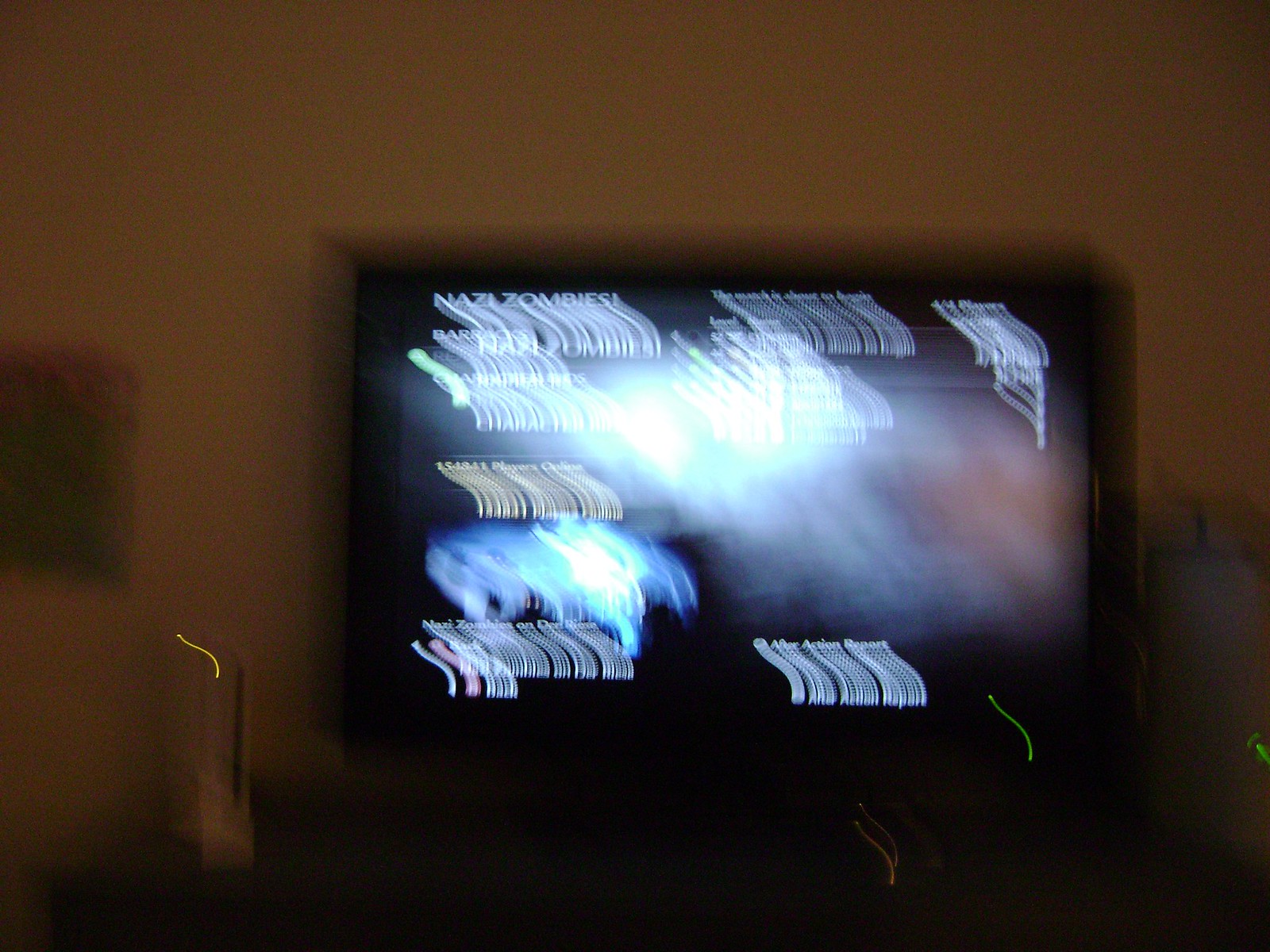The image is a horizontally oriented, blurry photograph capturing a dimly lit room with a television as its focal point. The TV screen, framed in black, is displaying an illegible array of words and images, though the phrases "Nazi Zombies" and "player choice" are discernible at the top. The television appears to be situated on a tabletop or TV stand. To the left of the screen, there's a vague outline of some sort of device, while to the right, another indistinguishable object can be seen. Behind the TV, the walls are a light color, likely whitish or beige, and are shrouded in shadows, contributing to the overall dark ambiance of the room. A picture is also faintly visible on the far left wall, adding a touch of decoration to the otherwise shadowy scene.